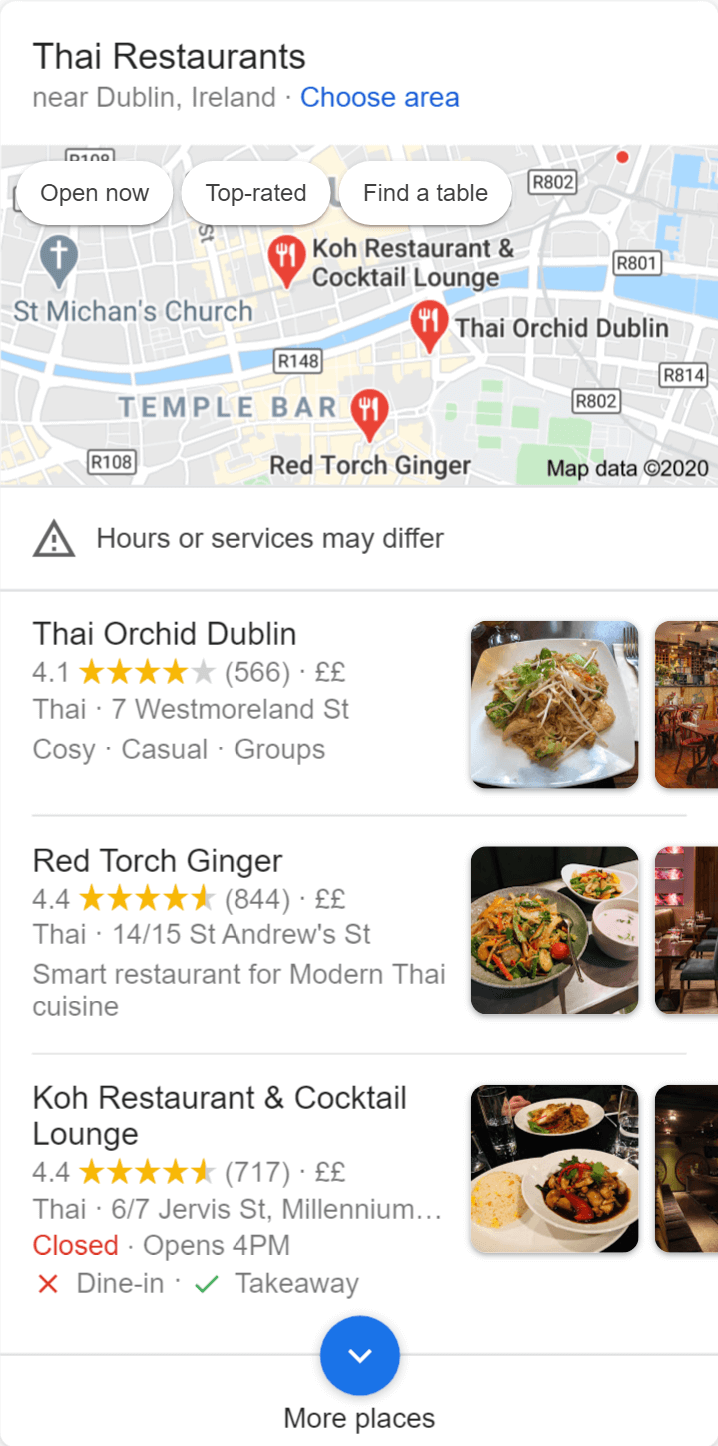### Websites - View on Mobile

**"Thai Restaurants Near Dublin, Ireland" Search Results**

*Screen Description:*

On a mobile device screen, the search heading reads "Thai restaurants near Dublin, Ireland." Below the heading, a blue hyperlink labeled "Choose area" is present. Directly beneath this, a 2020 map is shown, pinpointing various restaurant locations marked by spoon and fork icons.

Three filter options are available on the map interface: "Open Now," "Top Rated," and "Find a Table." A notification warns that hours or services may vary.

*Search Results Include:*

1. **Thai Orchid Dublin**
   - **Address:** Westmoreland Street
   - **Ambiance:** Cozy and casual
   - **Rating:** 4.1 stars
   - **Image Description:** A plate of traditional Thai food

2. **Red Torched Ginger**
   - **Address:** St. Andrews Street
   - **Rating:** 4.4 stars
   - **Image Description:** Thai cuisine served in a wok-style dish alongside a bowl of soup

3. **Coe Restaurant and Cocktail**
   - **Rating:** 4.4 stars
   - **Image Description:** A substantial bowl filled with a type of Asian soup

This clear, detailed compilation provides an easy-to-navigate layout for users seeking Thai dining options in Dublin via their mobile device.